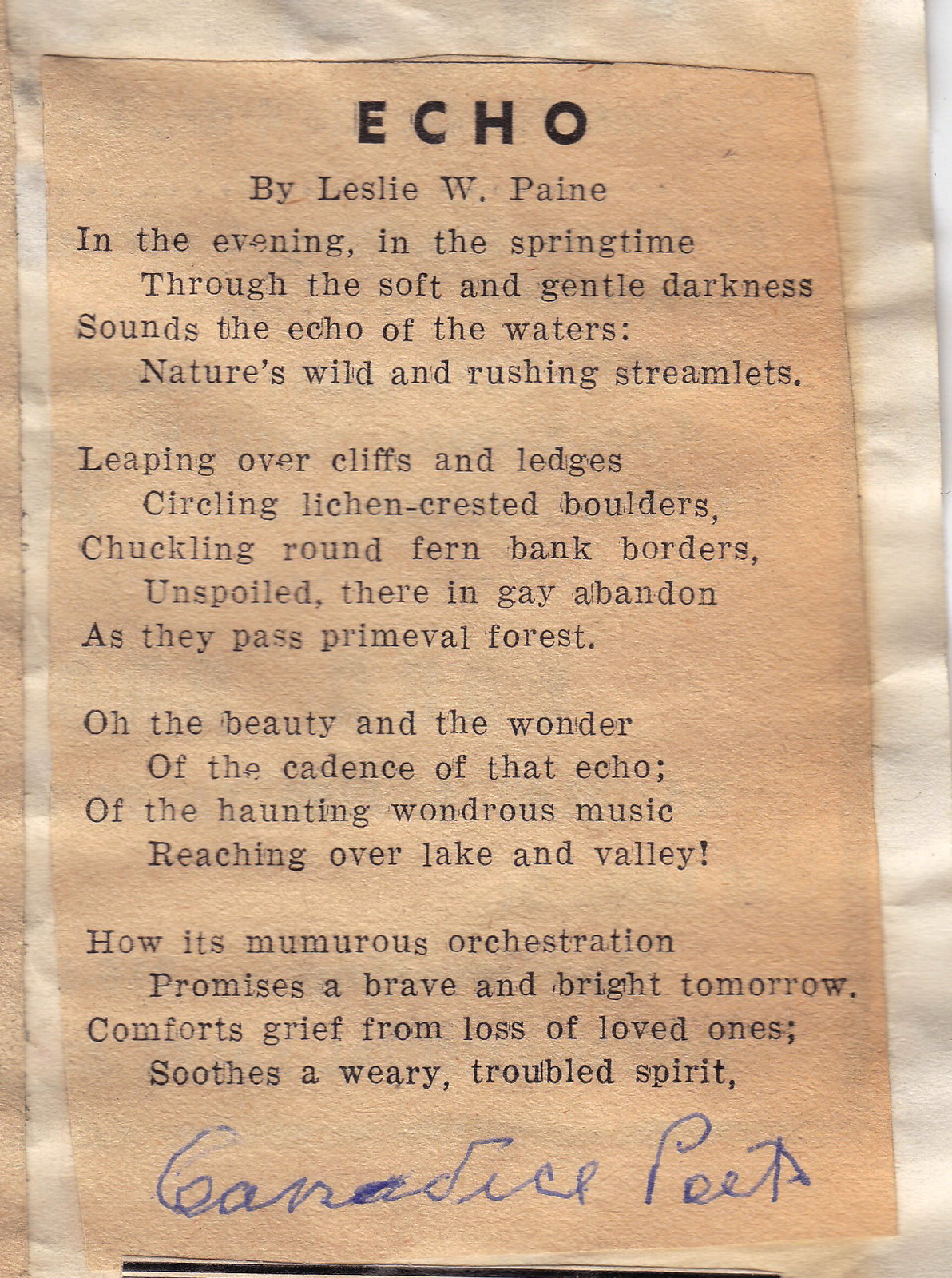The image depicts a poem titled "Echo" by Leslie W. Payne, printed on a light brown, possibly aged piece of paper. The title "Echo" is prominently displayed in bold black text, while the rest of the poem is typed in smaller black font. The poem reads: "In the evening, in the springtime, through the soft and gentle darkness sounds the echo of the waters, nature's wild and rushing streamlets, leaping over cliffs and ledges, circling lichen-crested boulders, chuckling around fern bank borders, unspoiled there in gay abandon as they pass primeval forest. Oh, the beauty and the wonder of the cadence of that echo, of the haunting wondrous music reaching over lake and valley. How its murmurous orchestration promises a brave and bright tomorrow, comforts grief from loss of loved ones, soothes a weary troubled spirit." At the bottom, there is a signature in blue ink that reads "Candace Pete," suggesting a personal touch or dedication.